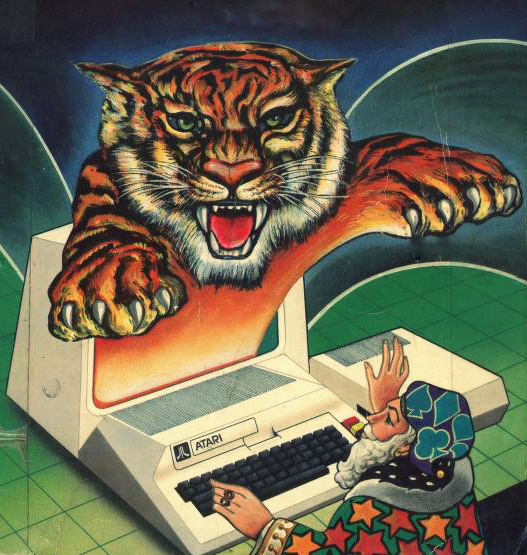In this captivating image, a person dressed as a whimsical wizard is depicted with great detail. The wizard is adorned in a vibrant green coat, embellished with a multitude of orange and red stars, with the top section of the coat being distinctively white. Atop their head sits a classic, curved wizard hat in a rich blue hue. Intriguingly, the hat features a green spade with white borders and a central diamond, as well as a clover.

To the right, the wizard’s hand is positioned near a green countertop, which is patterned with multiple squares. Adjacent to the countertop, there appears to be a gray plastic device, likely a scanner or printer. The scene becomes more fantastical with a tiger leaping out of a computer screen positioned in front of the figure. The computer, labeled "Atari," has a black keyboard with numerous keys. The screen vividly displays an orange backdrop from which the tiger emerges. The tiger, depicted with photorealistic detail, has white fur, prominent paws, an open mouth revealing sharp canines, and piercing green eyes. Its whiskers are clearly visible, adding to the lifelike depiction. Behind the tiger, the screen background transitions into a swirling blue area that adds to the dynamic energy of the scene.

The wizard, who has a large white beard and rings on their fingers, is enraptured by the scene unfolding on the computer screen. The overall composition marries elements of magic and technology, creating an engaging and imaginative depiction.